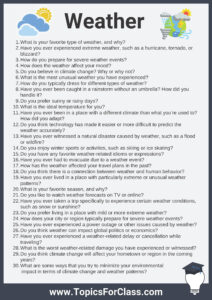The small, pixelated image is a graphical, text-based document with vivid weather-related illustrations. In the top left corner, two puffy clouds adorn the sky alongside a shining sun. The top right corner features an array of weather symbols, including a rain cloud, a tornado, gusts of wind, a sun partially obscured by a cloud, and a globe. The title, "Weather," is prominently displayed in large black text, capturing the theme of the document.

Beneath the title, a numbered bullet point list presents 30 weather-related conversation questions, such as "What is your ideal temperature?" and "Do you prefer sunny or rainy days?" This engaging list is designed to facilitate discussions about various weather preferences and experiences.

At the bottom of the image, a footer includes the URL "www.topicsforclass.com" alongside an icon of a light bulb wearing a black graduation hat, signifying the educational purpose of the document.